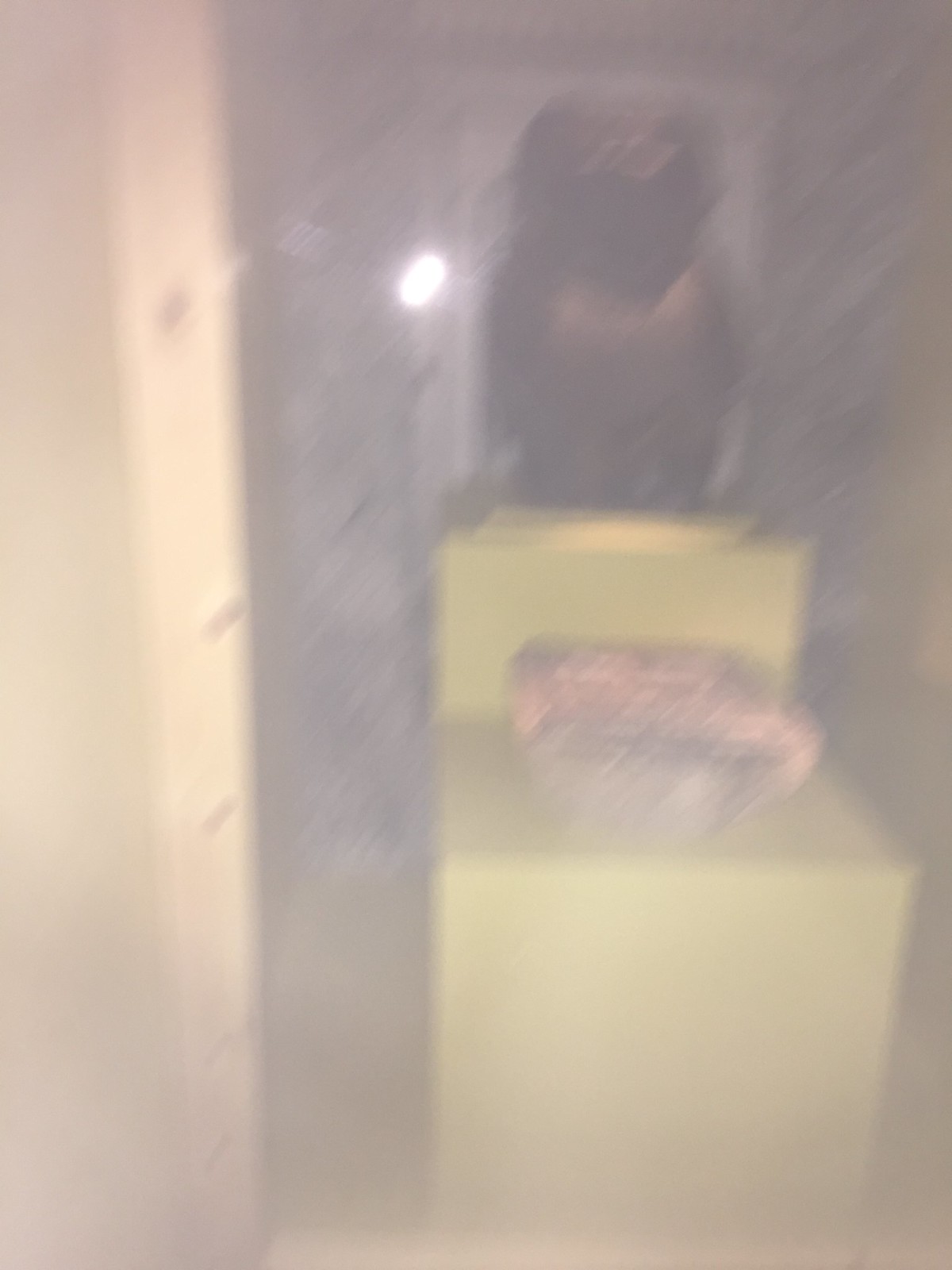This is a very blurry image, likely taken through a piece of glass or in a mirror due to the presence of multiple reflections. Central to the image is a dark chocolate brown statue that appears to be modeled after an Egyptian mummy, adorned with light brown accents. This statue is prominently placed on a small olive green washer, which has lighter green areas likely due to reflections from incoming light on the left. Additionally, there may be a stack of clothes on the washer, hinting at its functional context.

This washer and statue ensemble is set against a backdrop that features a white door with a matching white frame, situated within what seems to be a doorway. The background has a greyish, cement-like texture. Towards the top middle of the image, there's a clear reflection, possibly from a light source like a camera flash. This mirror or glass surface also has visible frame lines, suggesting the photo was taken through or at an angle with a reflective barrier.

The base supporting the statue and washer appears to be a yellow pedestal with sharp edges and 90-degree angles. Additionally, blurred and speckled white areas in the photo indicate a possible dirty lens or a poorly focused shot. On the right edge, there is a dark shape, potentially a coat or garment hanging, adding to the indistinct, cluttered nature of the scene. Overall, while the precise details are challenging to discern due to the blurriness, the image seems to depict a casual arrangement with both artistic and everyday elements in a visually complex setting.